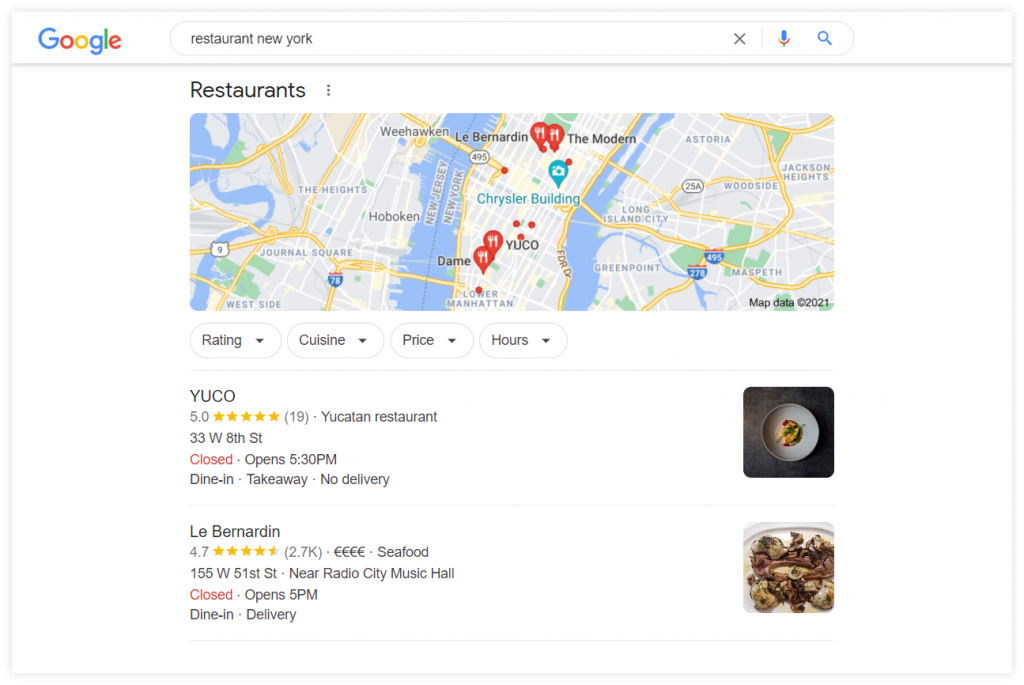The image is a screenshot from a Google search on a computer, displaying the search results for "restaurant New York." At the top of the results, the heading "Restaurants" is visible, followed by a list of restaurant options. The map of New York is prominently displayed, featuring several key elements: 

1. **Map Features:**
   - **Hudson River**: Clearly visible along with other waterways.
   - **Roads**: Highlighted in yellow.
   - **Green Land Areas**: Marked to indicate parks or other green spaces.
   - **Pins**: At least four red pins with fork and knife icons, indicating restaurant locations.

2. **Filter Options (Left Side):**
   - **Rating**: A drop-down menu for filtering results by rating.
   - **Cuisine**: A drop-down menu for filtering by type of cuisine.
   - **Price**: A drop-down menu for filtering by cost.
   - **Hours**: A drop-down menu for filtering by hours of operation.

3. **Restaurant Listings:**
   - **YUCO**:
     - **Rating**: 5.0 stars, based on 19 reviews.
     - **Cuisine**: Yucatan restaurant.
     - **Status**: Currently closed; opens at 5:30 p.m.
     - **Options**: Dine-in, takeaway (no delivery).
   - **Le Bernardin**:
     - **Rating**: 4.7 stars.
     - **Cuisine**: Seafood.
     - **Status**: Currently closed; opens at 5:00 p.m.
     - **Options**: Dine-in, delivery.

4. **Visuals**:
   - There are two images to the right of these restaurant listings, presumably showcasing the interiors or dishes of the respective eateries.

Overall, the detailed screenshot provides a comprehensive view of the search results for New York restaurants, including ratings, cuisines, operating hours, and service options.